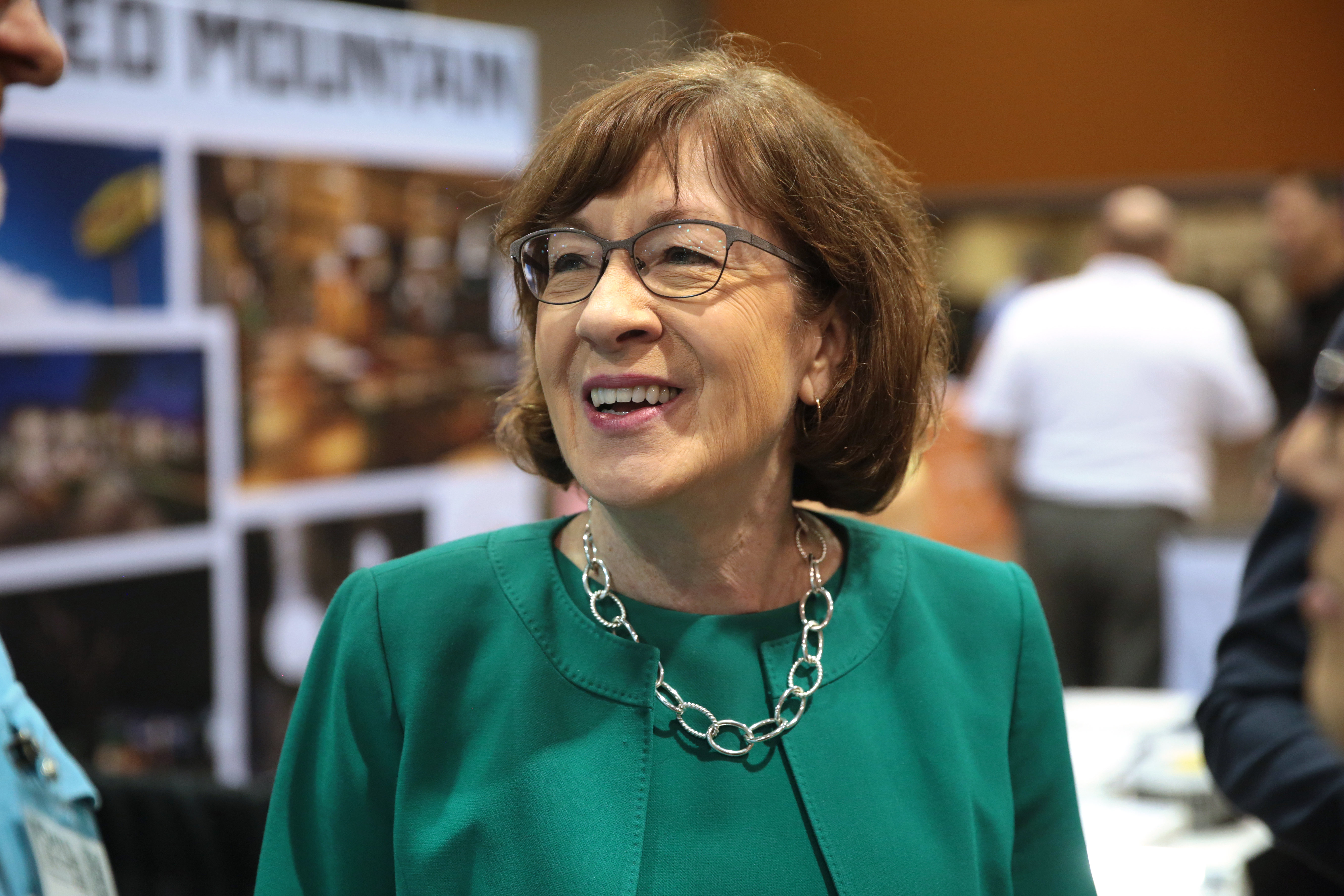In the image, an older woman is the focal point, characterized by her brown bob haircut with bangs and noticeable wrinkles around her eyes. She wears pink lipstick, gold earrings, and black-framed glasses. Her attire includes an emerald green top, a matching jacket, and a long, thick silver chain necklace. The setting appears to be a presentation or convention area, as indicated by the collage of images on a white poster board with black text in the background, partially readable as "mountain." To the left, a man with a partially visible face and shirt seems to be engaging with her, while another man with his back turned, featuring a noticeable bald spot, stands on the right. The background is filled with blurry figures and features a large white man in light and dark blue clothing. The overall scene is lively and bustling, with the woman appearing to be laughing and speaking with someone. The walls are brown, adding depth to the indoor event setting.